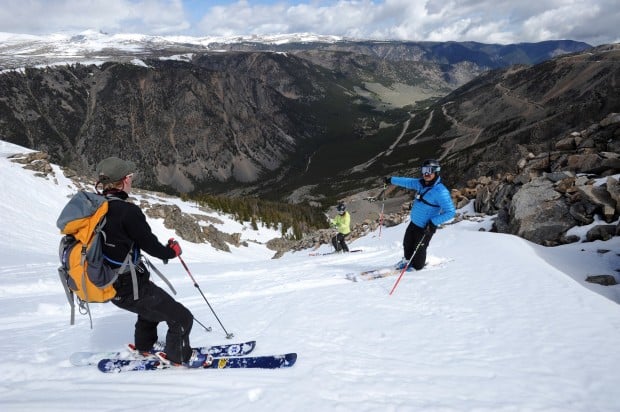In this detailed daytime photograph, three skiers are poised on a snowy slope with a vast mountainous background. The sky above is mostly cloudy, with small patches of blue peeking through. At the top of the image, one skier stands in an all-black outfit, wearing sunglasses, a grayish-green hat, and carrying an orange and gray backpack. He has his skis positioned sideways, secured in place by his planted ski poles. Slightly further down the slope, a skier in a blue puffy jacket and ski goggles points towards the valley below. The third skier, dressed in a lime green puffy jacket, is positioned even further down, appearing to wait for a signal from the others. The scene is layered with snow at the immediate area of the slope, transitioning to barren grass, dirt, and rock in the nearby valley. In the far distance, the peaks of distant mountains still hold snow, contrasting with the bare slopes closer to the skiers.